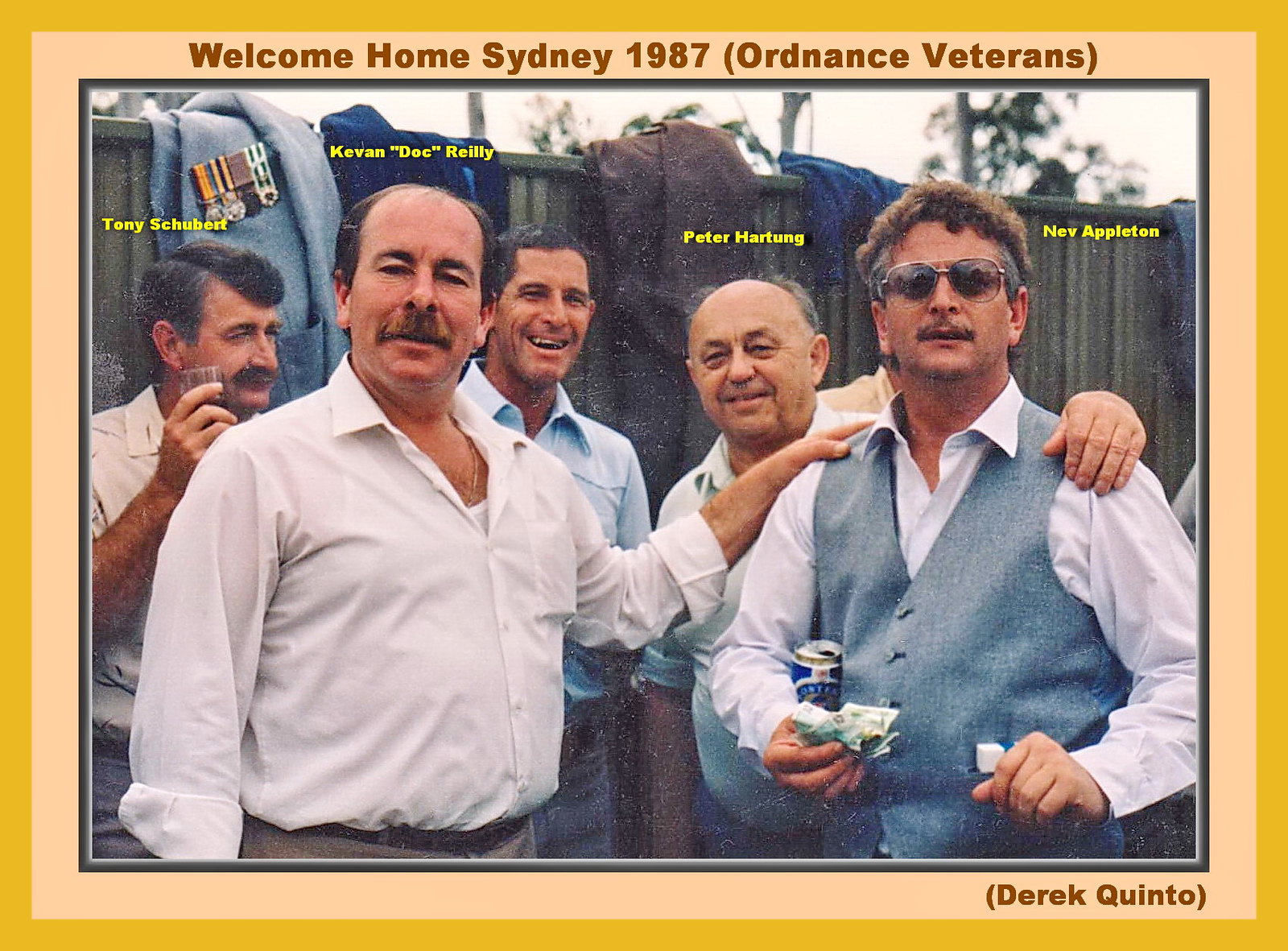This horizontally-aligned rectangular photograph is surrounded by a tri-border design: a light orange outer frame, an inner tan-colored border, and a gray inner frame. Between the picture and the frames, a light orange band contains the text in dark brown, "Welcome Home, Sydney, 1987 (Ordnance Veterans)." At the bottom right corner, it says "Derek Quinto." The image captures a group of five men identified by names in yellow text above their heads, appearing to enjoy a reunion or party.

From left to right:
- Tony Schubert, with a mustache and short brown hair, holding a shot glass.
- Kevin "Doc" Riley, a larger man in a long-sleeved white button-down shirt, bald on top with brown hair on the sides.
- Peter Hartung, partly obscured behind Kevin, smiling and wearing a light blue button-down shirt.
- A man in a collared shirt, identified as Peter Hartung. He has shorts, grayish-black hair around his bald crown, and is smiling.
- Nev Appleton, on the far right, wearing aviator sunglasses, a gray vest over his white collared shirt, holding cash in one hand and a beer can in the other, with cigarettes in his pocket.

The group stands in front of a wall that holds their overcoats, showcasing glimpses of the sky and tree branches above. The men, dressed in a mix of dress shirts and relaxed vests, appear to be enjoying themselves at a veterans' reunion, celebrating and reminiscing with drinks in hand.